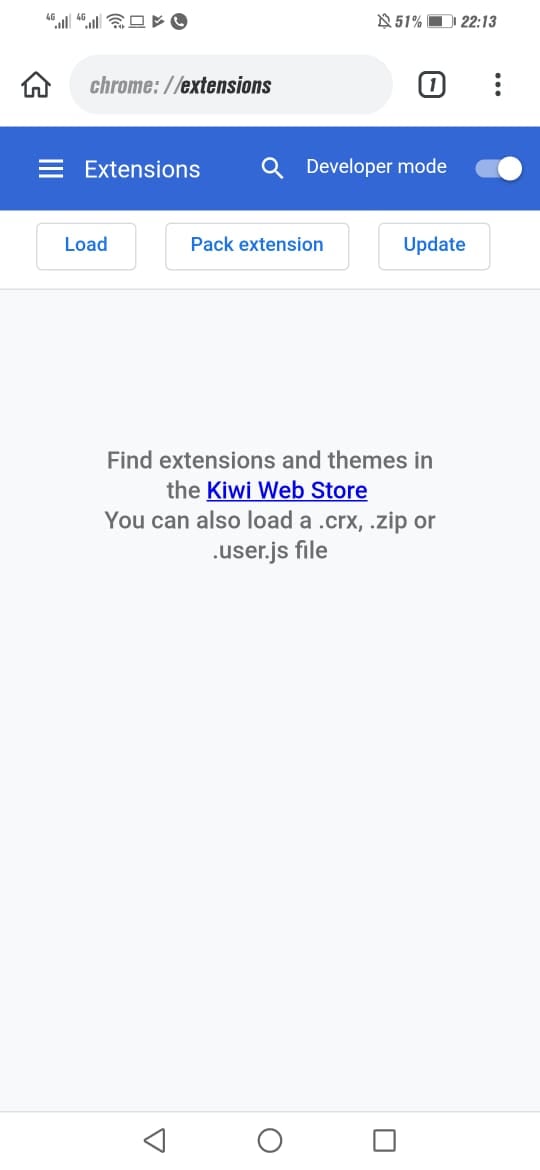A detailed screenshot of a mobile device display highlights various interface elements. At the top, the status bar is predominantly white, featuring a multitude of icons. There are two separate 4G icons, both showing strong reception with 4 out of 5 bars. Adjacent to these is a fully-lit Wi-Fi signal indicator. Additional icons include a monitor, a play button with a line through it, and a black circle containing a white phone icon. Progressing towards the right, there's a silent mode icon next to a battery icon displaying 51% charge, alongside a black battery level indicator. The time is shown as 22:13.

Beneath the status bar, the home screen displays a bubble for “chrome://extensions,” a numeral ‘1’ within a gray box, and three vertical dots. Below this, a blue bar contains three horizontal white lines and the word “extensions” in white. To the right of this is a white search icon, along with “Developer mode” in white text, and a selector button that is partially blue with a white circle.

Further down, a white bar presents three outlined icons in grayish-white boxes labeled "Load," "Pack extension," and "Update," all in blue. The remaining screen space is light gray, showcasing a prompt in gray text: "Find extensions and themes in the Kiwi Web Store." The "Kiwi Web Store" text is blue and underlined. Additional information mentions the capability to load files with extensions including .crx, .zip, or .user.js. Finally, at the bottom, there's a left-facing triangle icon, a circle, and a gray box icon.